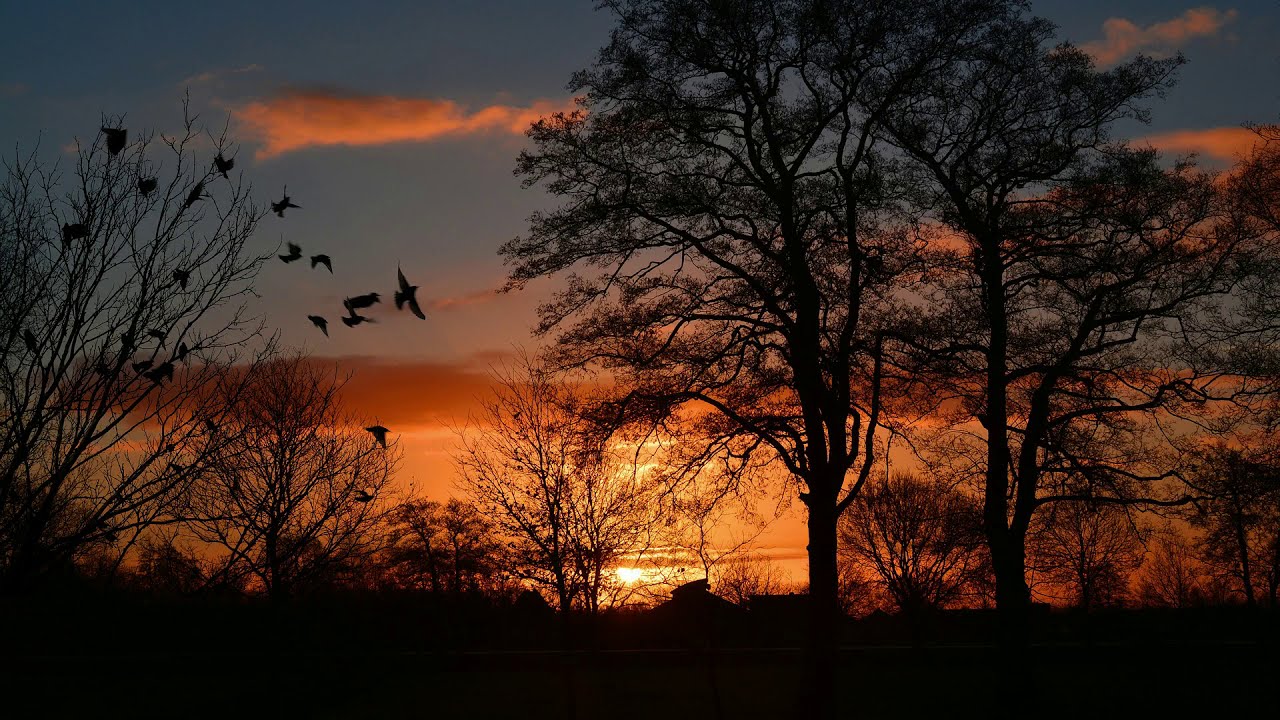In this serene sunset nature scene, the image captures the tranquil beauty of a park or natural area at sundown. Dominating the foreground are the dark, silhouetted forms of several large trees and some brush on the left. Wispy clouds tinged with blues, pinks, reds, and yellows scatter across the darkening sky, with the setting sun casting warm orange and gold hues that reflect off a distant waterline. Birds are depicted both perched in the limbs of the leftmost tree and in mid-flight, their silhouettes adding a dynamic element as some take off towards the right-hand side. Faint outlines of possibly two small houses can be detected at the center of the image, adding a subtle human touch to the otherwise purely natural setting. The overall composition conveys a peaceful, calming atmosphere, inviting viewers to appreciate the natural splendor of the moment.